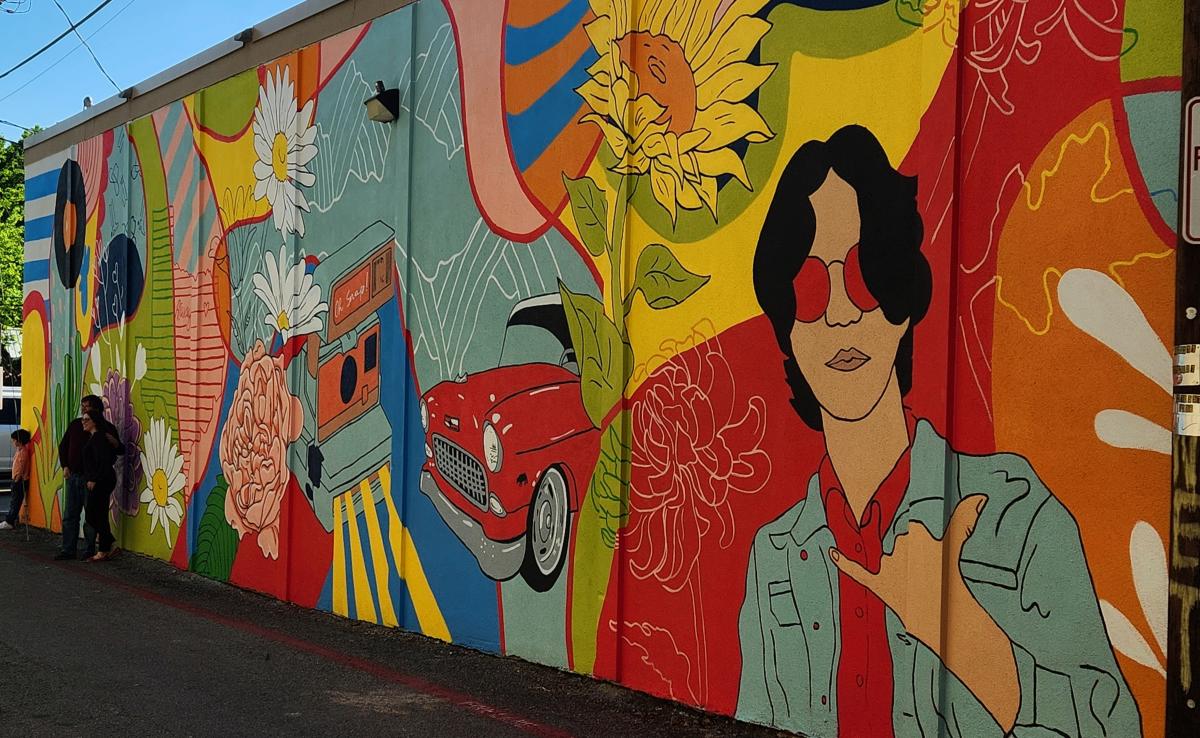The mural on the side of the building is vibrant and expansive, covering almost the entire wall and creating an eye-catching display that evokes a 'hippie' aesthetic. The prominent central figure in the mural is a tan man with dark hair, donning red sunglasses, a red shirt, and a denim jacket. He stands with his thumb and pinky extended in a classic "rock on" gesture. The background surrounding him is a psychedelic mix of orange, red, green, yellow, and blue tones. 

To the right of the man, there's a large sunflower, and right behind him, a bold red stripe adds to the vivid atmosphere. Adjacent to the sunflower, a red car with black wheels is depicted, which has been identified as an old Chevy with a white roof. Further to the left in the mural, there is an old video game console and clusters of white daisies with yellow centers, some looking like roses or peach-colored flowers. Additional white and vibrant-colored daisies are scattered around, enhancing the mural's floral theme.

In the upper left corner of the image, a small patch of blue sky is visible above the wall. At the left side of the mural, a man is standing next to a child, who is leaning against the colorful wall, likely both observing or participating in this artistic scene. The entire setting gives an impression of nostalgia mixed with exuberant artistic expression.